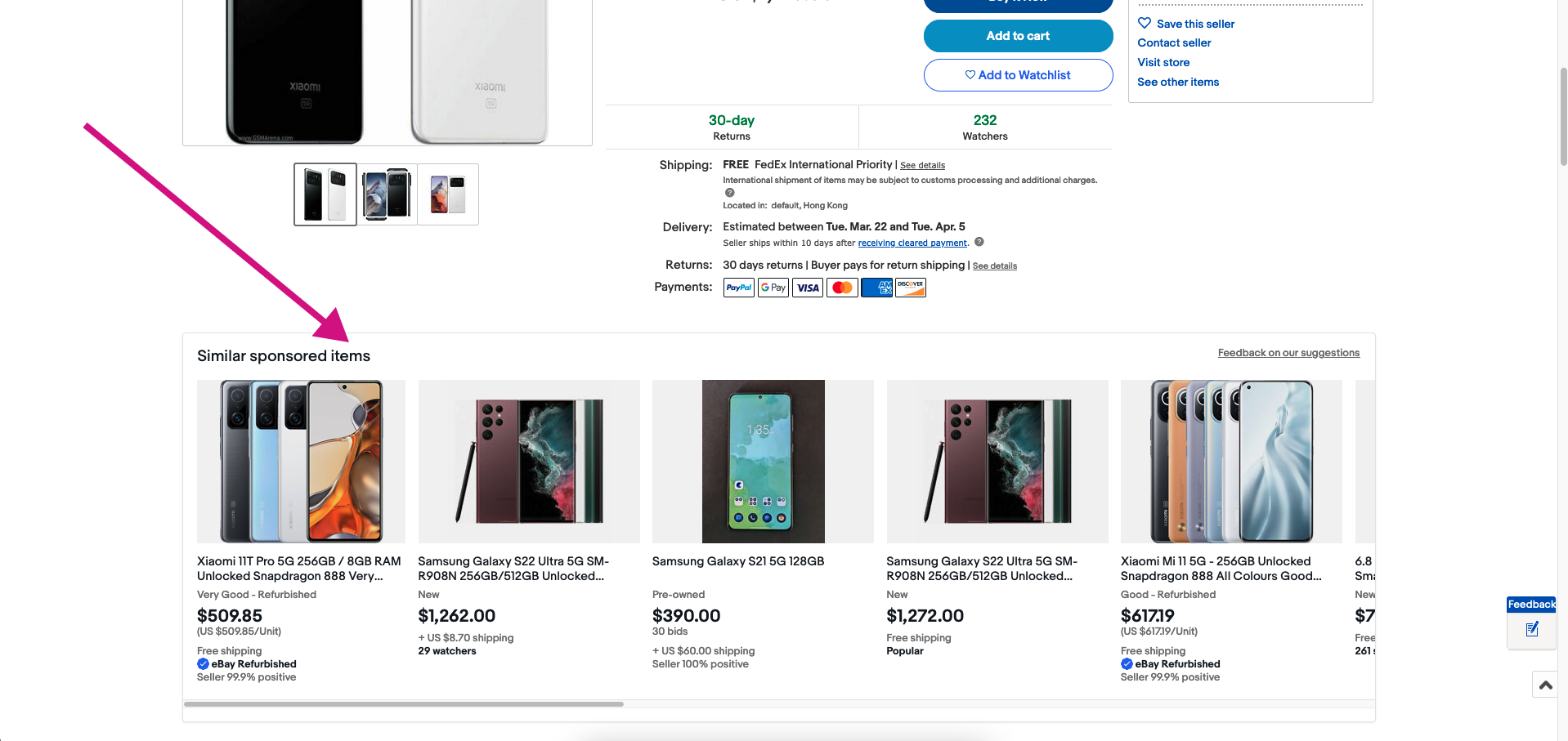A detailed caption for the screenshot:

"This screenshot, taken on a laptop or desktop viewing eBay, depicts a listing for a device resembling either a phone or an iPod, although the top portion is cropped and the item's price is not visible. Key interface elements are visible, including the 'Add to cart' and 'Add to watch list' buttons, a '30-day returns guarantee', and a note that the item has 232 watchers. The listing also mentions 'Free FedEx international shipping' with an estimated delivery window between March 22nd and April 5th. Multiple payment options are noted, including PayPal, Google Play, Visa, and MasterCard, among others. Below the listing, a section for 'Similar Sponsored Items' displays products such as Xiaomi phones, Samsung Galaxy models (including the S21, S22, and S22 Ultra), and a Xiaomi 256GB unlocked phone. The items have prices ranging from $390 to $1,262, and all appear to be available via auction."